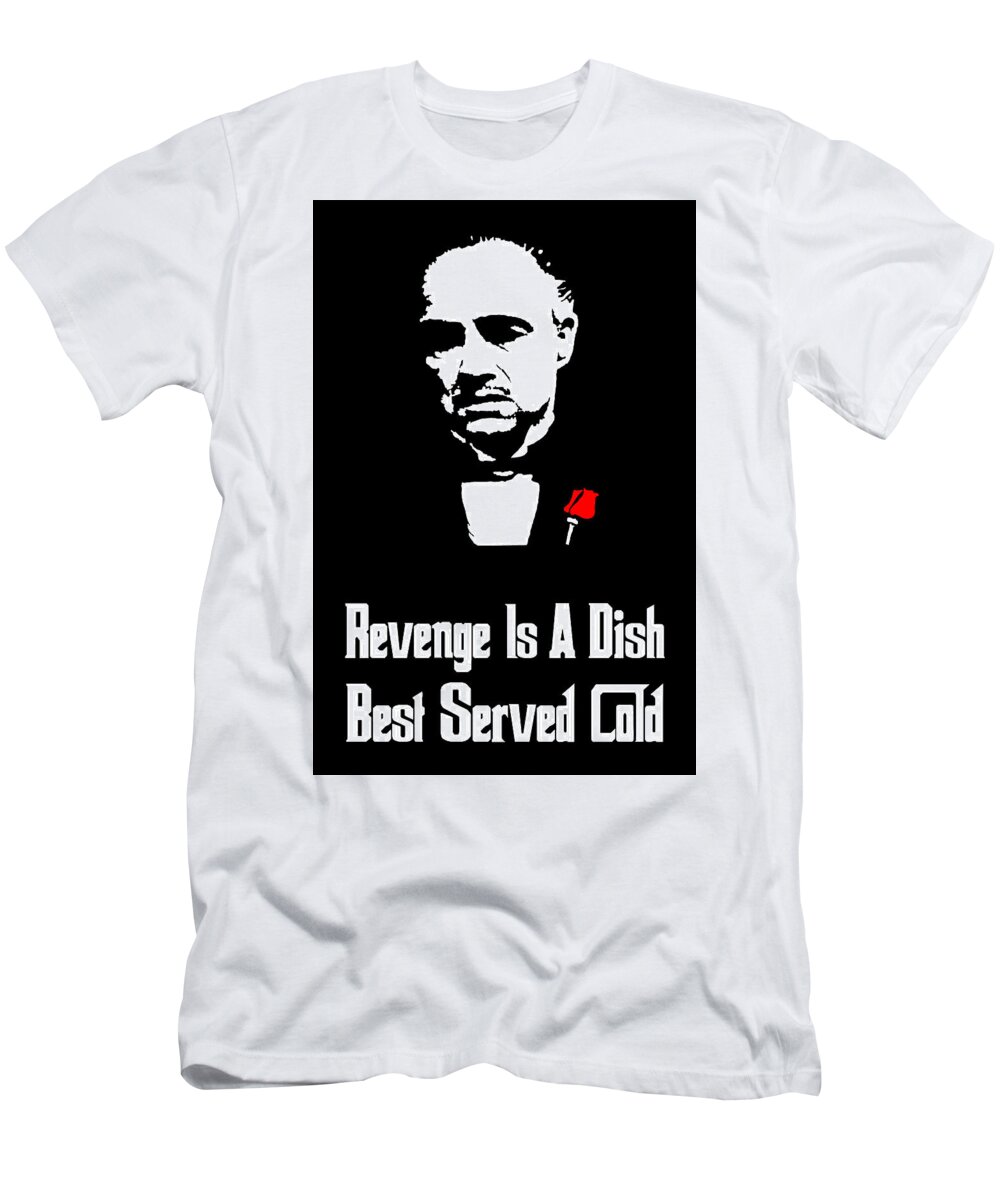This photograph captures a basic white, short-sleeved t-shirt, slightly wrinkled, adorned with a striking graphic design on the front. At the center of the shirt, a large black rectangle prominently features a black-and-white image of Marlon Brando as the Godfather. The character, appearing older and unamused, is depicted wearing a suit jacket with a distinctive black bow tie and a red rose on the lapel, the sole splash of color in the design. Beneath the image, in a font matching the iconic movie cover, the text reads, "Revenge is a dish best served cold." This t-shirt, conveying a classic and cinematic aesthetic, is a tribute to the legendary film.